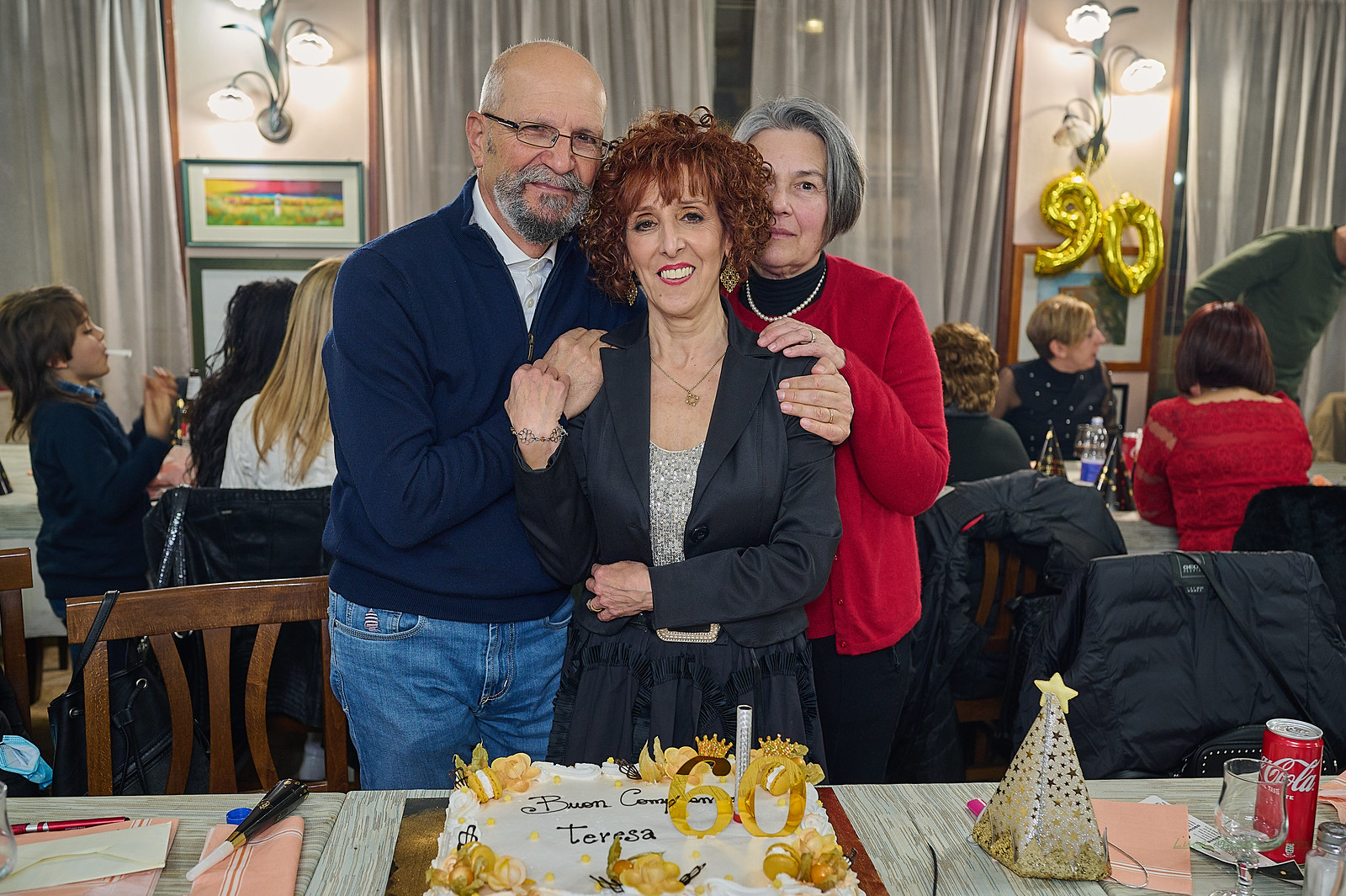The image captures a celebratory scene at Teresa's 60th birthday party. At the center of the picture stands a woman with crimped, short, brownish-auburn hair styled beautifully. She wears a striking amount of makeup, with vivid red lipstick highlighting her broad, straight-tooth smile. Her outfit includes a black blazer over a silver top, paired with a black skirt that features ruffled trim. A man and a woman, each with a hand on her shoulder, flank her. The man on her right wears a long navy blue zip-up hoodie over a white shirt, blue jeans, and sports a bald head with a gray beard and mustache combo, accented by thin-framed rectangular black glasses. On her left stands a woman with short gray hair, clad in a red, long-sleeved sweater with a dark undershirt, black trousers, and a pearl necklace.

In front of them lies a white sheet cake adorned with gold flowers, bearing the name "Teresa" and the number "60." The table also holds a variety of items, including pink napkins, a silver party hat with gold stars, a can of Coca-Cola, a salt shaker, and a wine glass. Background elements include gold balloons spelling out "90" (potentially accidentally inverted), and glimpses of seated guests further emphasize the event's lively atmosphere.